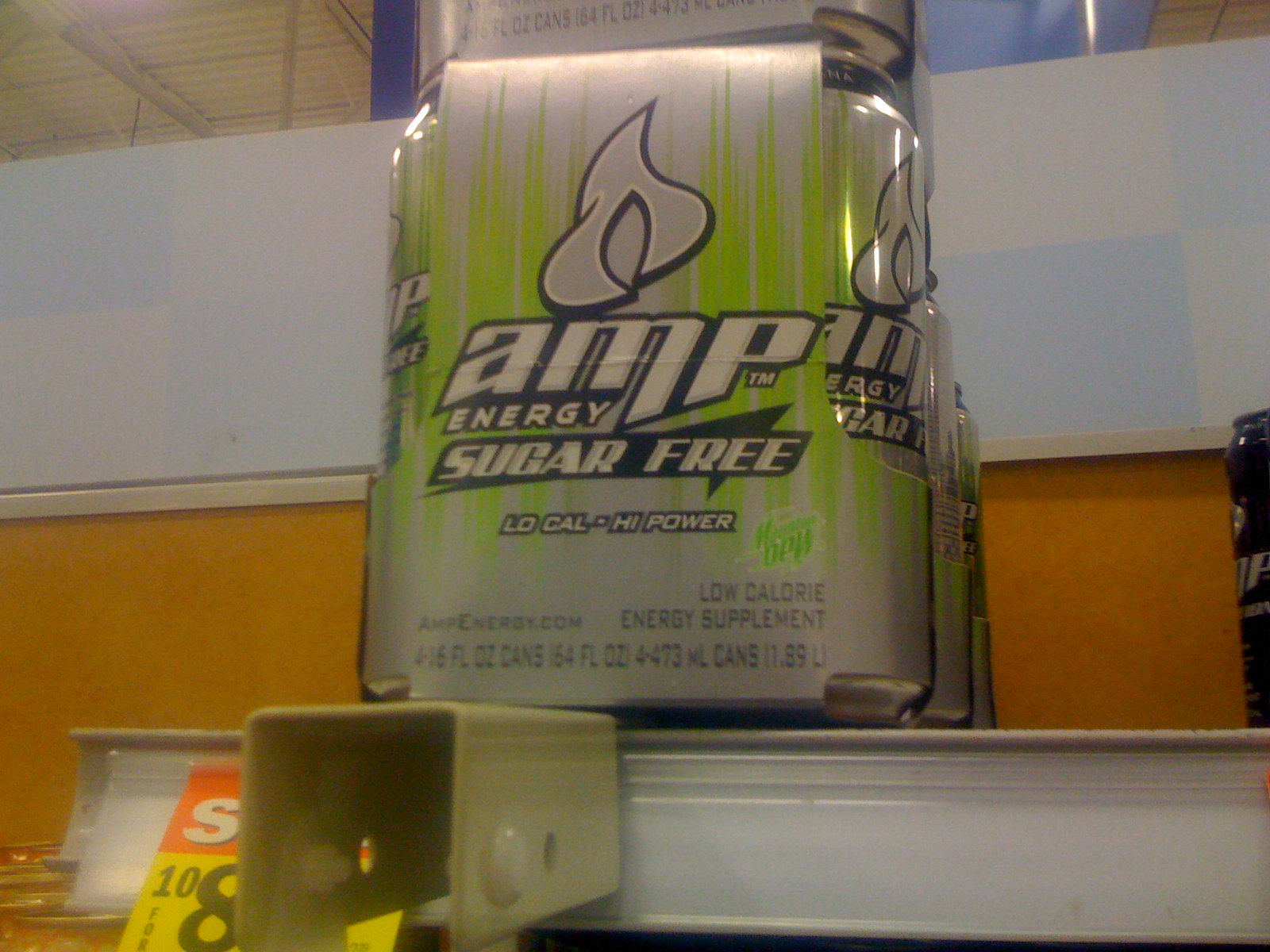The image depicts a close-up of an AMP Energy Drink multipack, likely from the mid-2000s. The packaging prominently features four 16 fluid ounce silver cans with green vertical lines and the brand "Amp energy." The cans are partially visible through the paper wrapping, which markets the drink as sugar-free, low-cal, and high-power. The multipack rests on a store shelf, under a red and yellow sale sticker that partially displays the price, starting with an 8. The shelf has a distinctive white and blue checkered pattern on the back wall and brown elements below. Some additional text on both the packaging and the price sticker is obscured by the angle of the photograph.